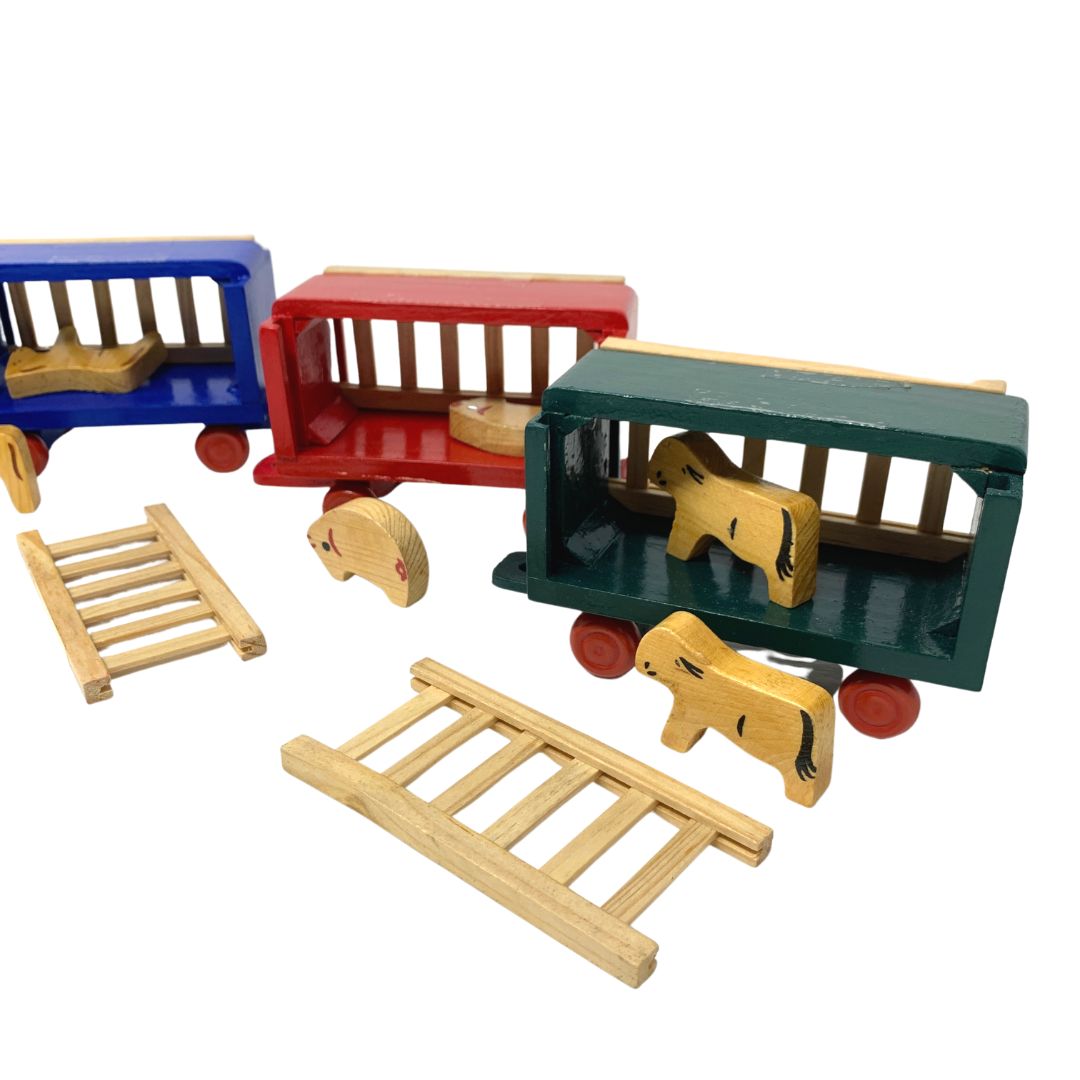The photograph depicts three toy train cars positioned on a stark white surface against a white background, giving the illusion that they are floating in a void. The train cars, each crafted from wood and featuring red wheels, are arranged sequentially from left to right in blue, red, and green colors. Each car is equipped with removable light brown wooden railings that serve as cage bars; these side panels are laid next to the cars within the scene.

The blue train car, positioned on the left, holds a brown wooden animal resembling a horse with a black tail, lying down inside. The red train car in the middle contains a rounded pig-like wooden creature tipped over inside. Additionally, another pig-like figure, partly colored with red and black, stands outside the cart. The green train car on the right features a goat-like creature standing upright within it. Furthermore, outside this cart, there is another animal that looks like a cow. The wooden animals are simple, carved shapes with minimal markings that hint at their identities, adding to the charming, handcrafted aesthetic of the toys.